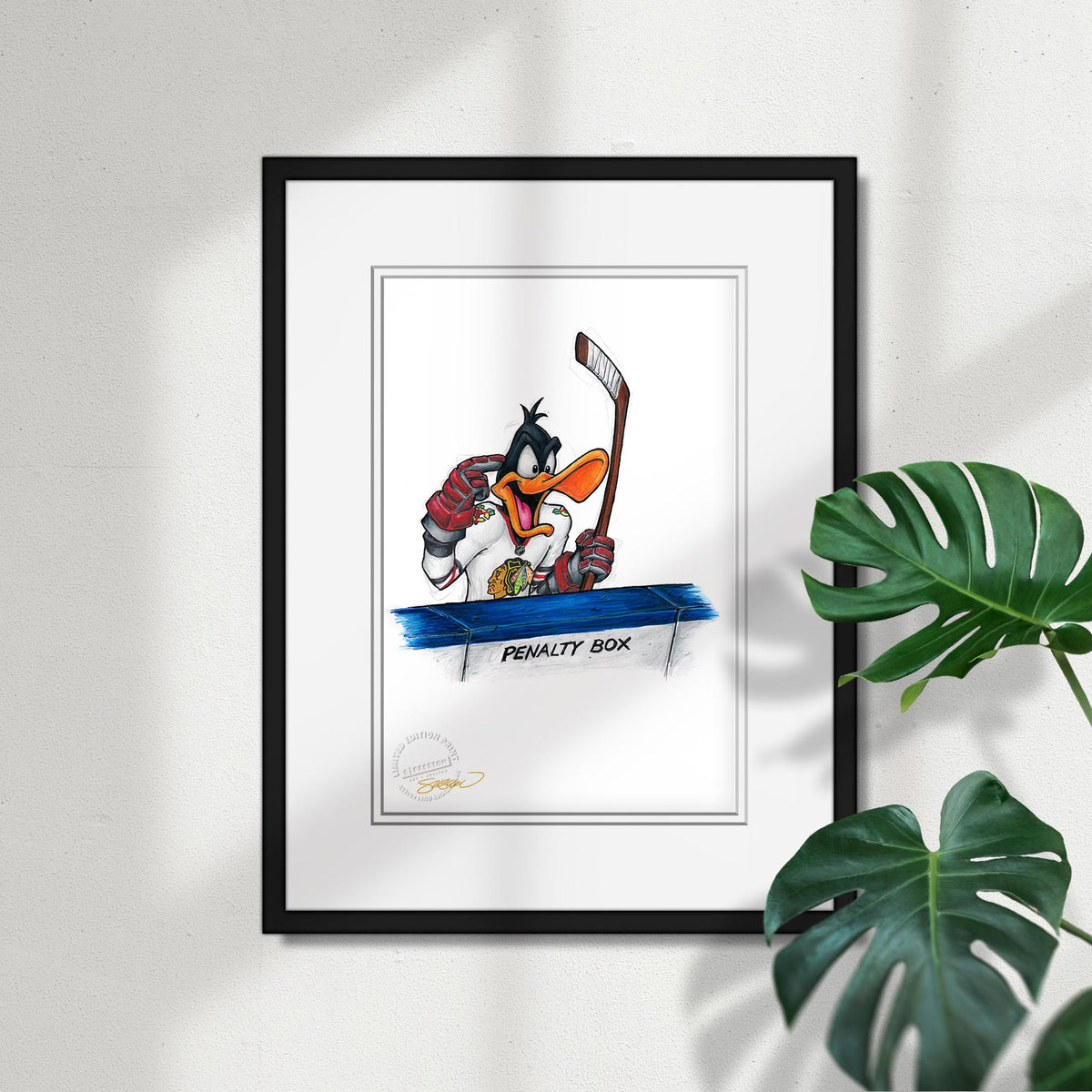This detailed painting captures Daffy Duck dressed as a hockey player, situated in a penalty box. Daffy is wearing a white jersey adorned with a black hawk logo, and big red gloves; his expression is one of irritation, as he appears to be yelling and pointing forward with his right hand, his mouth open to reveal his pink tongue. He holds a brown hockey stick with white tape at the end. The penalty box, marked with the words "penalty box" in black lettering on a blue rail, only shows Daffy from the waist up, with the top of the railing and a bit of the front visible in gray.

The painting is framed with a black border and two white mats, and is displayed on a white wall. Sunlight streaming through a window casts squares of light across the wall, enhancing the overall setting. Large green leaves from a plant on the right side cast additional shadows, some overlapping the painting slightly. A watermark or signature in gold ink is noticeable in the lower left corner of the artwork.